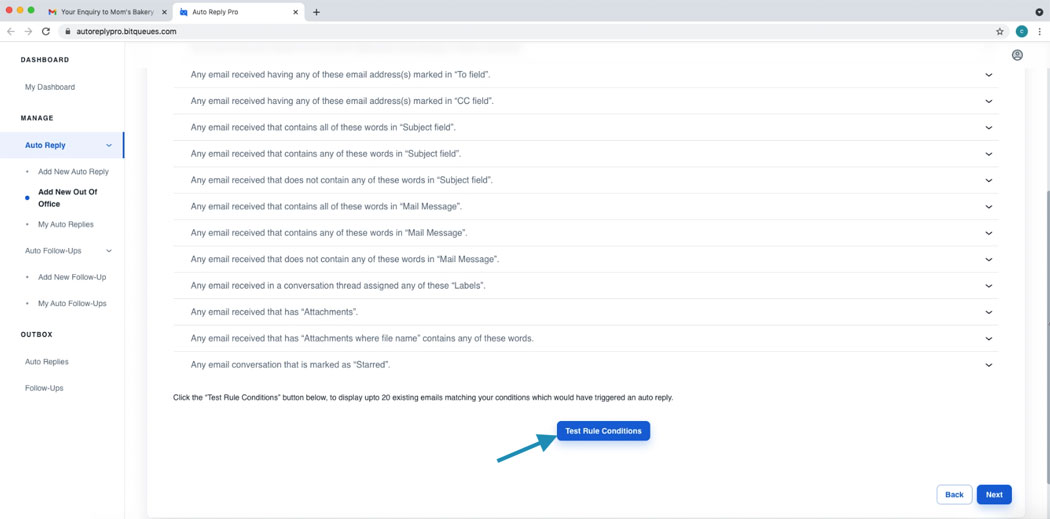The screenshot displays a compact user interface, making text readability challenging due to its small size. On the left side of the screen is a vertical menu. At the top of the menu, the word "Dashboard" is clearly visible, and beneath it reads "My Dashboard." The subsequent section in the menu is labeled "Manage," and directly under that is "Auto-Replay," which appears to be expanded.

Upon expanding the "Auto-Replay" section, we see the option to "Add New Out of Office," located to the right of the menu. This section contains a list, which partly reads, "Any email received having any of these email..." followed by some text in quotes that is difficult to discern due to its small font size.

At the bottom center of this section, there is a button labeled "Test Rule Conditions," with an arrow pointing towards it, indicating its significance or suggesting the next action to take.

This detailed description presents an organized view of the elements visible within the screenshot, albeit the tiny text poses some challenges for full clarification.